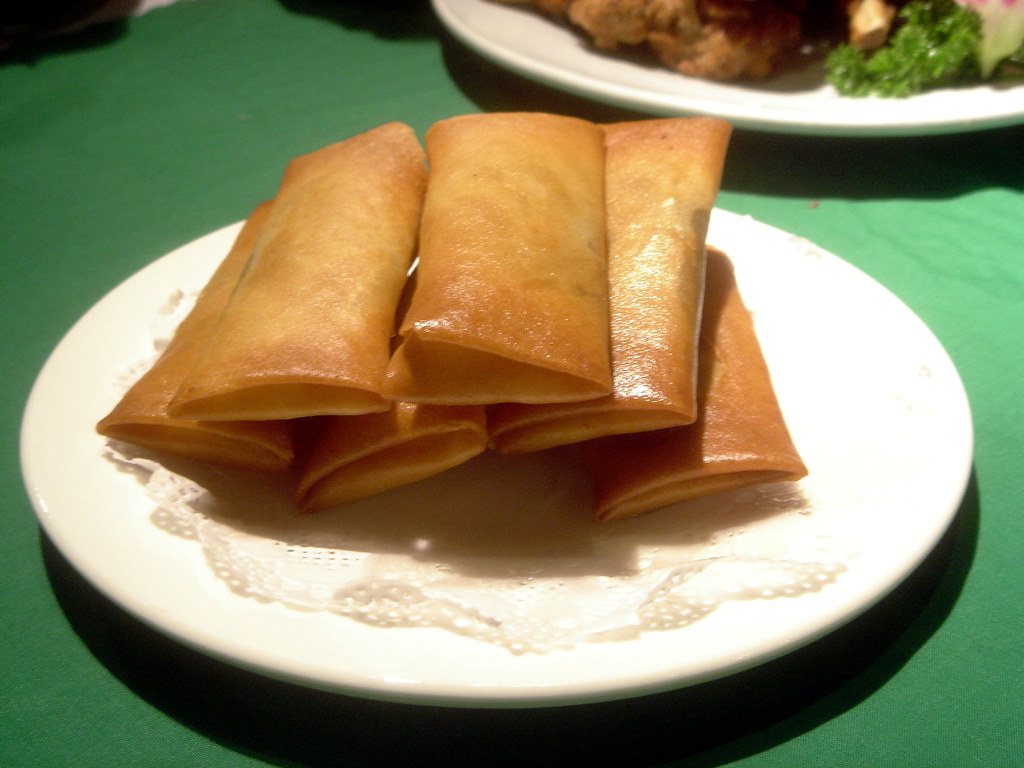In this detailed image description, we see a close-up, rectangular, color photograph with a landscape orientation, capturing a central white plate adorned with a delicate white lace doily. On the doily, arranged neatly, are six golden-brown, rectangular spring rolls with shiny surfaces, suggesting they may have been brushed with egg wash or deep-fried. These flattened, envelope-like rolls give the impression of being nearly empty. The plate is situated on a green tablecloth that serves as the background. Beyond the central plate, there's another partial view of a plate of food, featuring green items, possibly some broccoli and other vegetables, along with some meat. The focus remains heavily on the spring rolls in the foreground, emphasizing their glossy texture and arrangement.